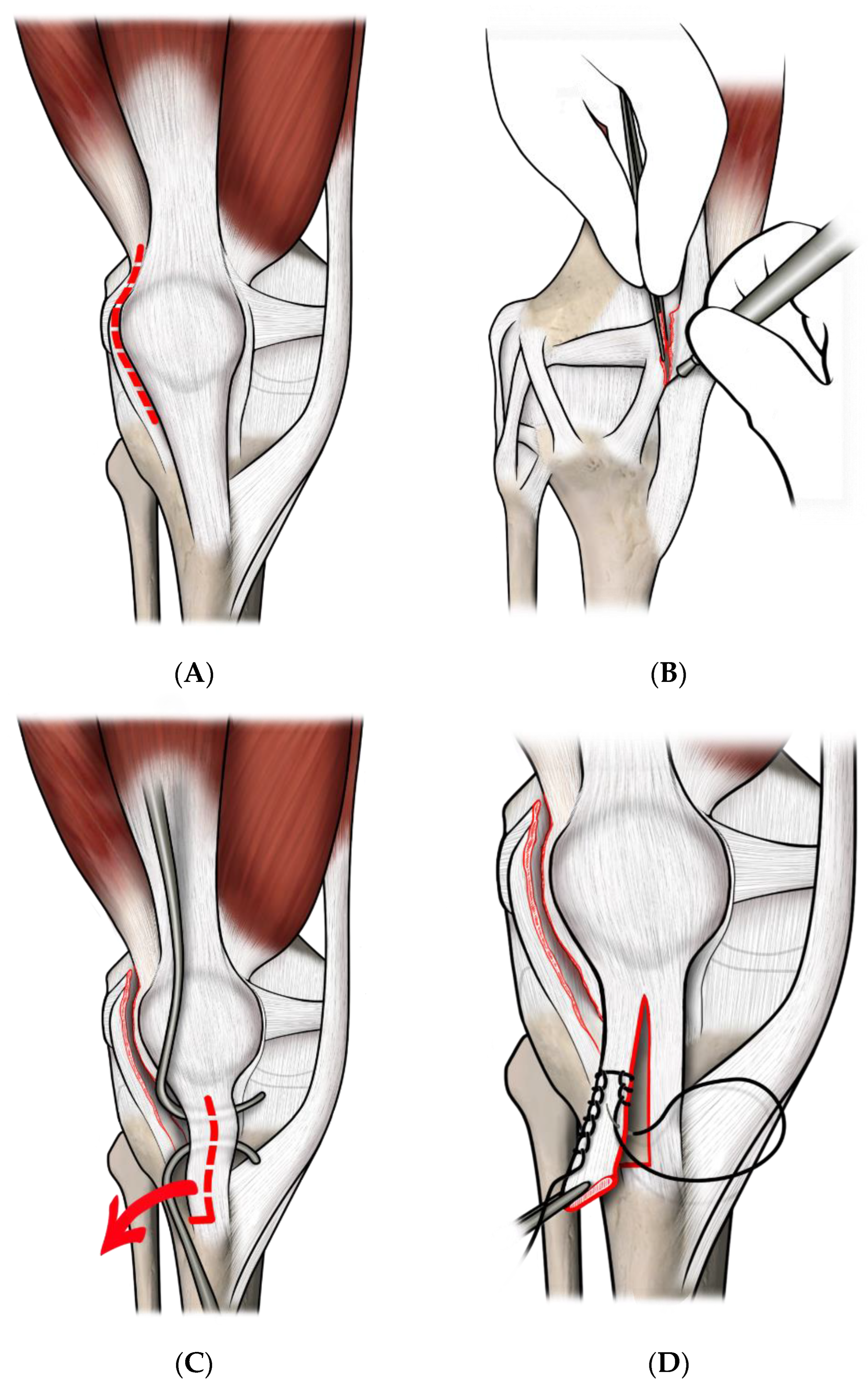This detailed black and white and colored instructional drawing, set indoors, includes four labeled figures (A, B, C, D) of a knee joint, rendered in black and white with accents in orange, brown, and red. Each drawing is of identical size and organized in a two-by-two grid.

**Figure A** illustrates the upper portion of a knee, featuring red muscle tissue, a bone, and a knee cap. Red dotted lines indicate where an incision is to be made. **Figure B** shows the hands of a surgeon using a scalpel to cut along the marked red line adjacent to the bone. **Figure C** describes the process post-incision, detailing further surgical steps. **Figure D** mirrors the Figure A diagram but with an added red line running down the bone under the knee cap, indicating a completed incision. It also shows black sutures applied to the side of the bone beneath the knee cap. The images collectively present a detailed step-by-step visual guide for a knee surgery.